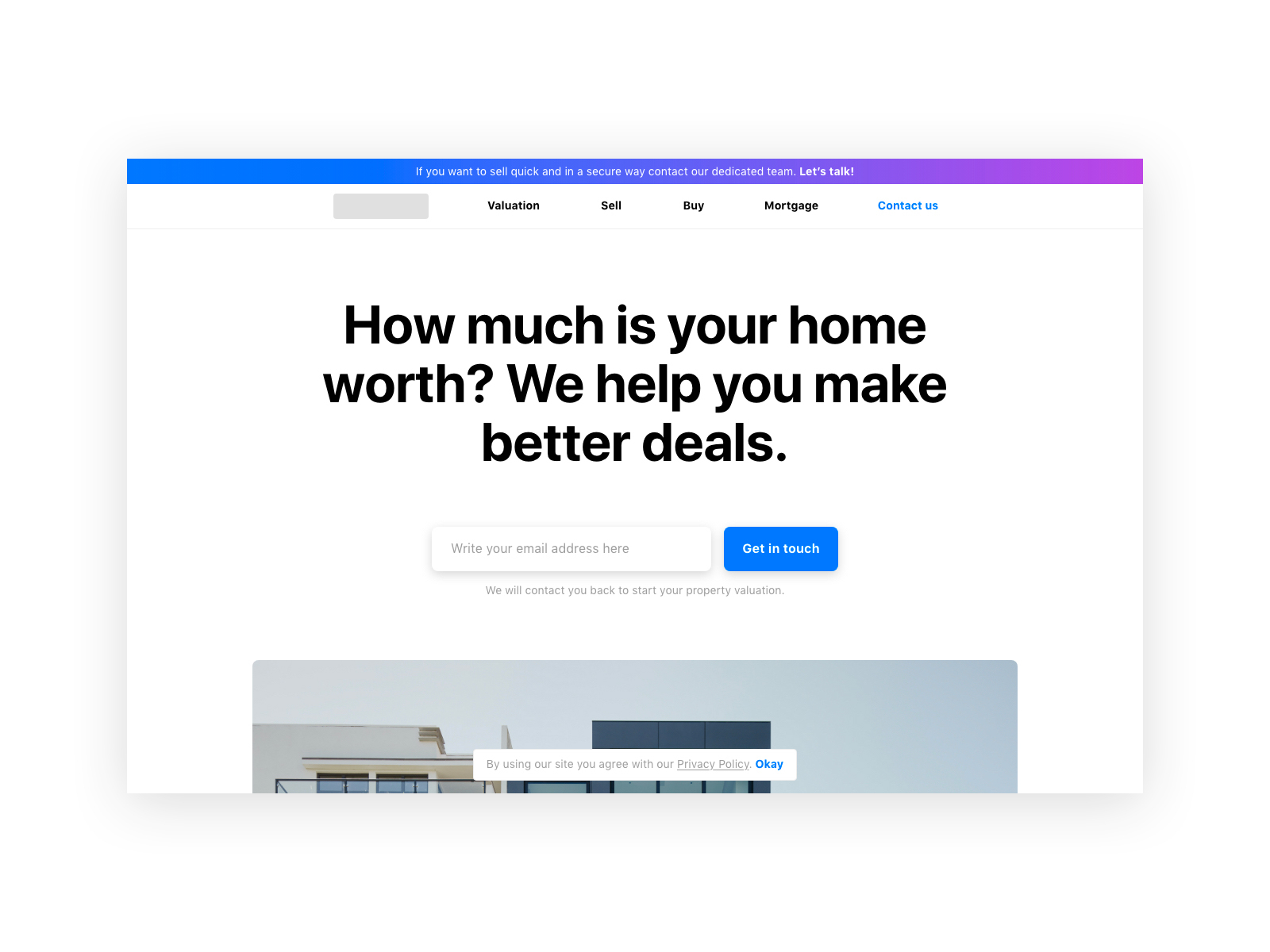This image showcases a website with certain elements obscured. The name or logo of the website is intentionally grayed out, thus hidden from view. The top of the page features a prominent long rectangle banner that transitions in color from blue on the left, to purple, then to pink as it extends to the right. Text within this banner reads, "If you want to sell quick and in a secure way contact our dedicated team," followed by a bolded call to action, "Let's talk!"

Below this colorful banner, the website's menu bar is displayed against a white background. The left side where the website's name or logo would typically appear is covered by a gray rectangular box. The menu bar features black text links labeled "Valuation," "Sell," "Buy," and "Mortgage," with the "Contact Us" link highlighted in blue on the far right.

The central header of the webpage asks in large black text, "How much is your home worth? We help you make better deals." Directly below this header, there is an input field prompting users to "write your email address here." To the right of this input field is a prominent blue button with the text "Get in touch" centered within it. The overall design is clean and emphasizes user engagement and contact.